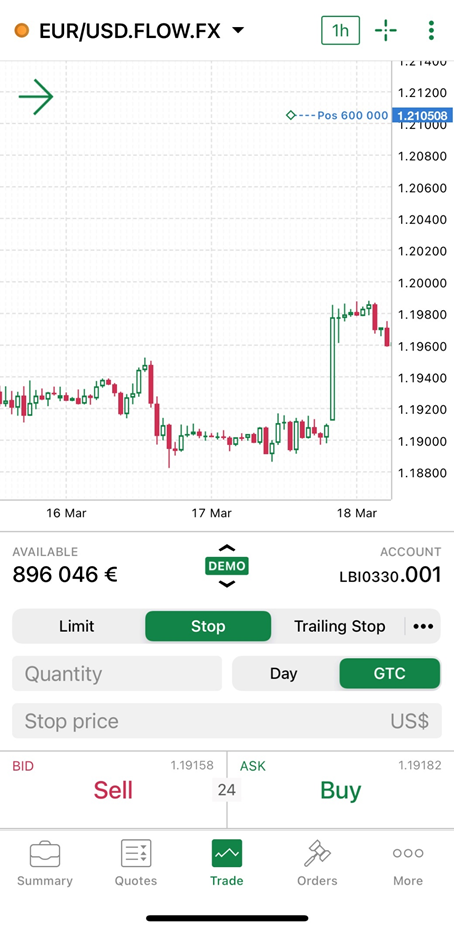This image is a detailed screenshot from a trading application, focusing on the EUR/USD (Euro to US Dollar) currency pair. The chart at the center of the image is set to a one-hour (1H) time frame, meaning each candlestick on the chart represents one hour of trading activity. The candlestick chart visually represents the price movements over this period, with green candlesticks indicating price increases and red candlesticks signifying price decreases.

At the top, the header prominently displays "EUR/USD," clearly indicating the currency pair being monitored. The application's interface likely includes several other trading features and data points, although they are not all highlighted in the provided description.

Beneath the chart, there is a section showing the available balance of 896,046 Euros in a demo account, designated as "LBI0330.001." This substantial balance suggests that the user is trading in a simulated environment, a feature commonly offered by trading platforms to allow beginners to practice and test different strategies without the risk of losing actual money. This demo setting is especially useful for honing trading skills and gaining familiarity with the platform's functionalities.